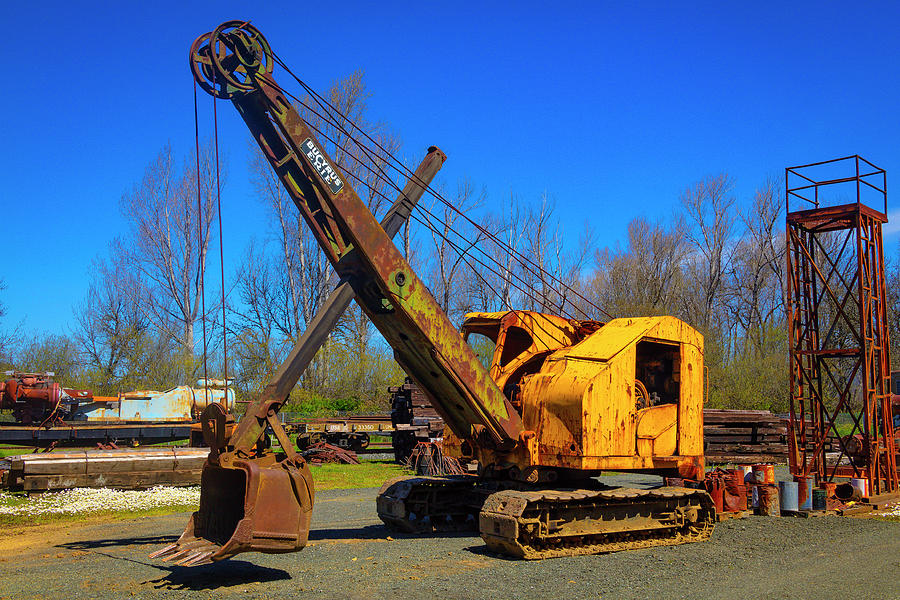This outdoor photograph captures an industrial construction scene centered around an old, rusted yellow crane situated slightly to the right of the image. The crane's body, compact and nearly cubic with some curves, sits on olive-green tank-like tracks, casting a shadow beneath. The crane's arm, made of rusty metal, extends from its front at a 45-degree angle, reaching almost twice the height of the crane's body. A scissor-shaped element of the crane angles downward in the opposite direction, positioning the bucket close to the ground, almost horizontally. The setting is an industrial yard with a gravel pavement. In the background to the left, there are trees without leaves, some other rusty industrial equipment, and what appears to be old train tracks with flatbeds. To the right of the crane, the image shows a pile of various metal and plastic containers and a rusty, two-story climbing platform structure that looks like scaffolding. The sky above is vividly blue, giving a bright and oversaturated feel to the overall photograph.